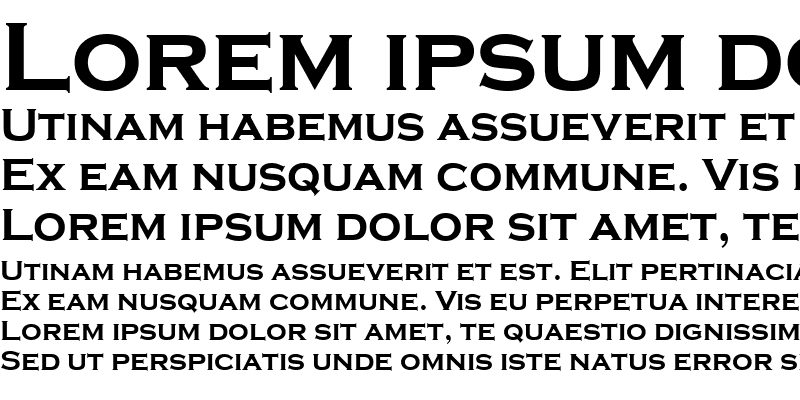The image depicts digitally-created text on a plain white background. The black text is structured to evaluate different font sizes and styles. At the top, a large, bold heading begins with "LOREM IPSUM D," but it cuts off. Below that, there are three lines of medium-sized text, followed by four lines of smaller text. These lines contain filler phrases from the Latin placeholder text commonly known as "lorem ipsum." The sequence of the text shows a gradual decrease in font size and boldness, demonstrating how the fonts and headings might appear. Some lines are partially cut off, adding to the sense that this image is a test or mockup for evaluating typography.